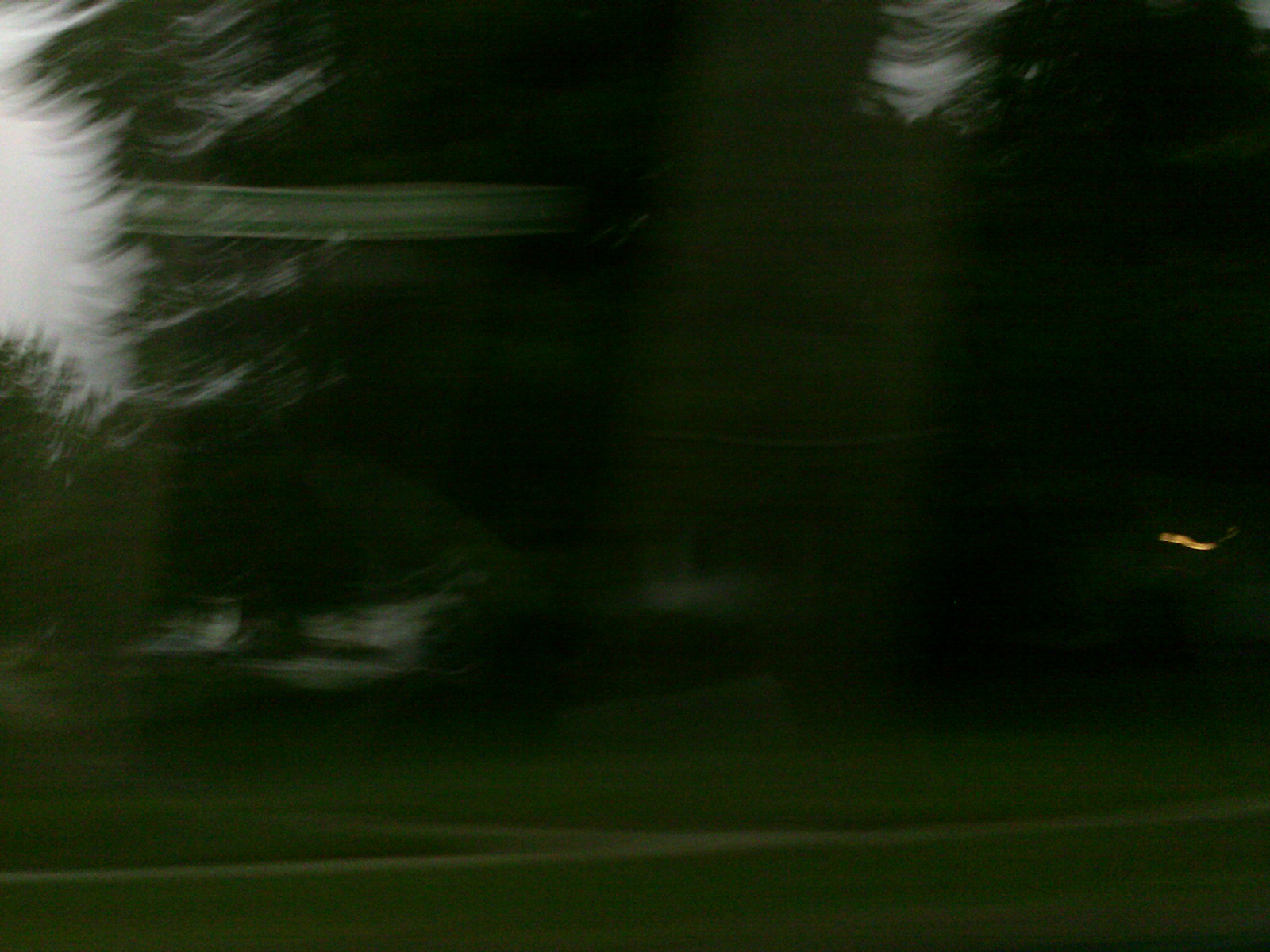A motion-blurred photograph, likely taken from within a moving vehicle, captures the fleeting scenery of a road framed by reflections on a glass window. The bottom of the image shows a flat, gray roadway with a prominent yellow line running through it, indicating the dividing line. Above the road, a backdrop of dark, dense trees dominates the scene. There are faint reflections on the road's surface, including a wide vertical line that runs straight down. On the left side of the image, a blurred green and white sign is barely discernible. The ambient light suggests the photo was taken during sunset, with the entire scene enveloped in the warm, fading light of dusk.